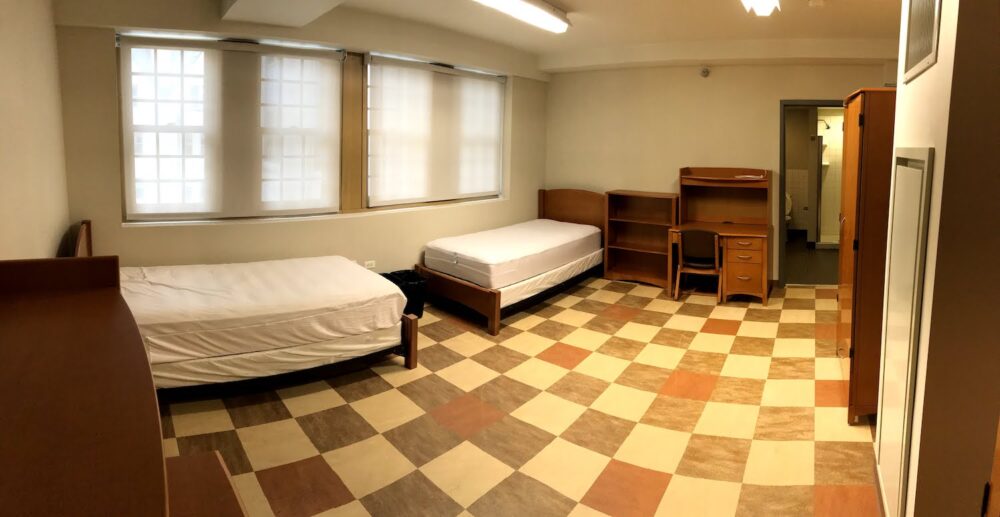This image depicts a sparse, dual-occupancy room that could be mistaken for either a hospital room or a hotel room. The floor is covered in a distinctive checkerboard pattern comprising shades of mustard, brown, cream, and black. The spacious room houses two twin-sized beds with wooden headboards and footboards, positioned such that their feet face each other from opposite ends of the room. Both beds are bare, with mattresses but no linens. The room's walls are painted white and bathed in ample light, both natural and fluorescent. On the left wall, multiple windows are covered with translucent, blurry shades, diffusing the light that streams in. The right wall features a short, three-shelf bookcase, a wooden desk, and a chair. Additional furnishings include a large wooden dresser or closet. In the background, there is a glimpse of what appears to be a bathroom, indicated by the visible edge of a toilet and a shower room. The overall color scheme is neutral, emphasizing the room's emptiness and clinical feel.